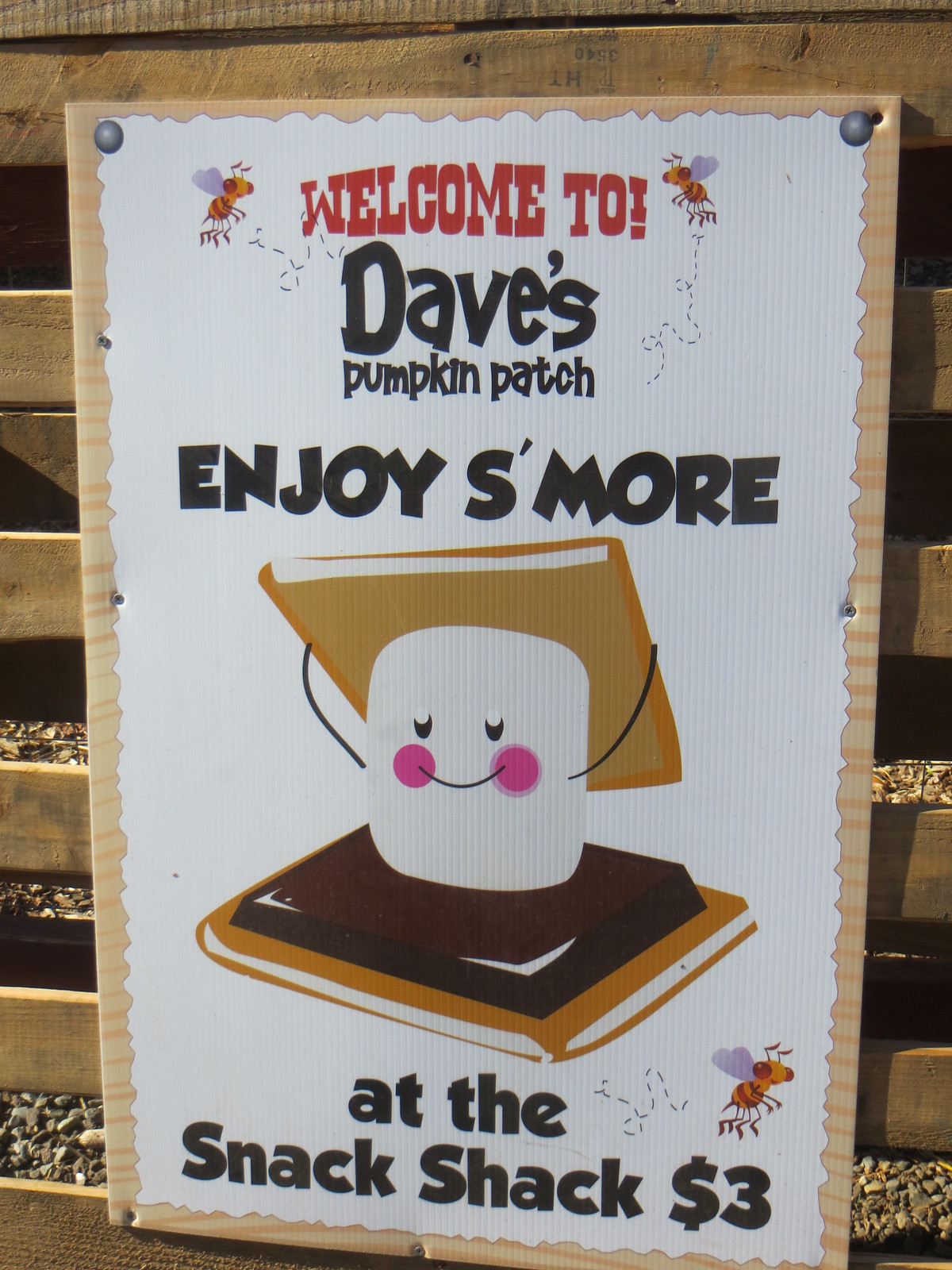This is a detailed photograph of a sign affixed to a wooden fence, with some gravel and dirt visible in the background. The sign itself has a beige border and a white, slightly cardboard-like background. At the top of the sign, there are two illustrated bees flanking the text "Welcome to Dave's Pumpkin Patch" written in red and dark stylized fonts. Below this, the sign reads "Enjoy s'more at the Snack Shack. $3.00." Between the phrases "enjoy s'more" and "at the Snack Shack," there is a charming cartoon illustration of a smiling s'more with black eyes and pink round cheeks. The s'more consists of a smiling marshmallow positioned between two graham crackers and a layer of chocolate, with the top graham cracker held above the marshmallow's head. Additionally, a bee is illustrated flying right above the price of three dollars. The overall composition of the sign is inviting and festive, aimed at welcoming visitors to Dave's Pumpkin Patch and enticing them to enjoy a treat at the Snack Shack.